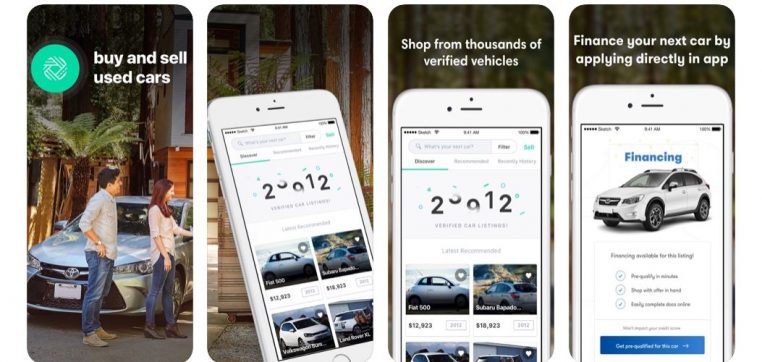This series of four smartphone-shaped screenshots visually narrates an advertising campaign for a car buying and selling app. 

In the first panel, a young couple, consisting of a male and female, stands proudly in front of a sleek silver Toyota sedan, symbolizing a successful purchase facilitated by the app. 

The second panel features a side view of a smartphone displaying four diverse cars for sale, highlighting the app's wide range of options. 

The third panel captures a front-facing screenshot of the app, where the number "23912" is prominently displayed with digits animated to resemble slot machine reels, suggesting the vast inventory available to users. 

In the final panel, the focus is on a pristine white SUV with the word "Financing" emblazoned above it, emphasizing the app's financing options. 

At the top, white text instructs users: "Finance your next car by applying directly in-app," reinforcing the convenience and comprehensive services offered by the app.